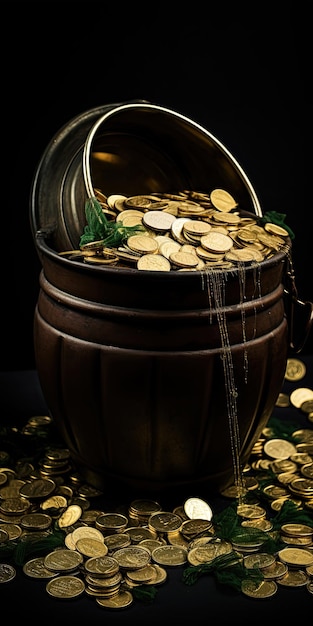The image depicts a dark brown barrel overflowing with an abundance of gold coins, so full that the coins are spilling out and scattering across the floor. The close-up view highlights the intricate details of the unique, non-American coins. A mysterious silver element is present around the barrel, adding to its distinctive appearance. The barrel itself has two noticeable ridges and appears to be partly encased in another dark brown container. On the left side, a small green plant peeks out among the coins, while a pale, stringy material dangles from one side. The background is a stark black, accentuating the vivid contrast with the shimmering gold coins and the deep brown of the barrel, creating a striking visual effect.